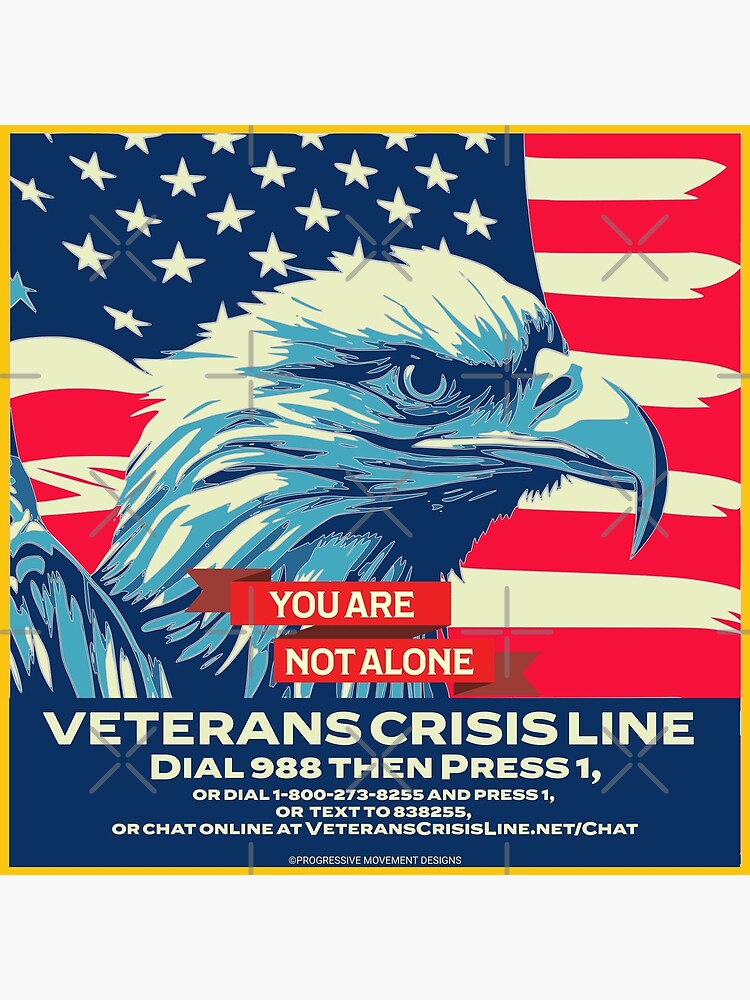This image features a detailed painting of the head of a fierce-looking bald eagle, characterized by white feathers and a beak shaded with blue. The eagle is prominently centered against an artsy depiction of the American flag, with white stars on a blue background positioned in the upper left corner, and red and white stripes on the right. The background is accented with a gold border, enhancing the patriotic theme. Overlaying this imagery are significant text elements in bold white letters: a red text box that reads "You are not alone" and a blue text box at the bottom that provides essential information for the Veterans Crisis Line. The instructions are: dial 988 and press 1, or dial 1-800-273-8255 and press 1, or text to 838255, or chat online at veteranscrisisline.net/chat. This powerful composition, labeled "Progressive Movement Designs," serves as an important advertisement for veteran support services.